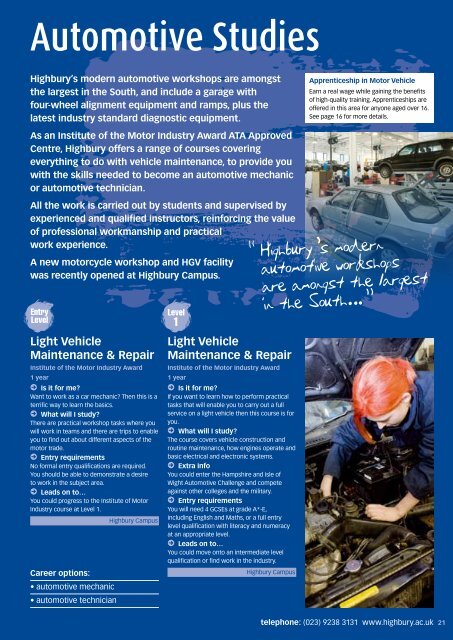The image features a female mechanic with red hair working diligently beneath the engine of a car, illustrating hands-on learning in automotive studies. The backdrop is rich blue paper with prominent white text headlines, emphasizing Highbury College's cutting-edge automotive workshops. Highbury prides itself on having some of the largest and most modern facilities in the South, featuring four-wheel alignment equipment, ramps, and state-of-the-art diagnostic tools, all endorsed by the Institute of the Motor Industry (IMI) ATA. This brochure highlights the diverse range of courses offered, including entry-level and Level 1 Light Vehicle Maintenance and Repair, designed to provide students with the practical skills and professional expertise necessary to pursue careers as automotive mechanics or technicians. The workshops are overseen by experienced instructors, ensuring high standards of workmanship. Highbury also recently expanded its amenities to include a new motorcycle workshop and a Heavy Goods Vehicle (HGV) facility. The program promotes earning while learning through quality apprenticeship opportunities available to anyone over 16, providing an excellent pathway to gainful employment in the automotive industry. For more details, prospective students are encouraged to call 023 9238 3131 or refer to page 16 of the prospectus.